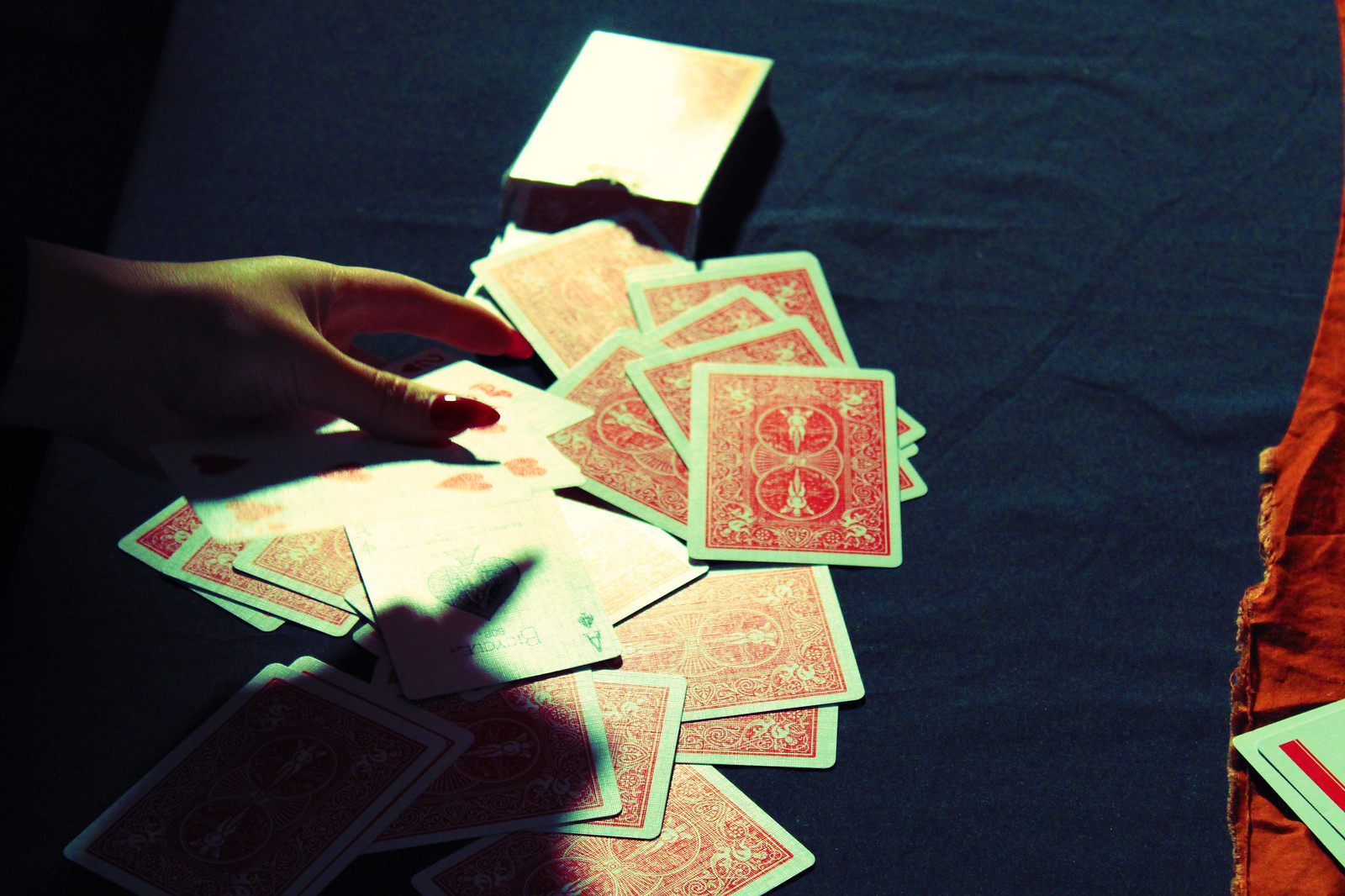In a dimly-lit photograph, a dark navy blue tablecloth is draped over a flat surface. A woman's hand, adorned with red nail polish, rests elegantly amidst a scattered array of playing cards. Some cards lie face down, while others display their intricate designs. A cardboard box, presumably for the cards, is also visible. A harsh white light beams down, illuminating the cards and the woman's hand, and creating a stark contrast with the surrounding dark areas. The intense glare of the light washes out the colors of the cards, making the illuminated area much brighter compared to the dark border surrounding the scene.